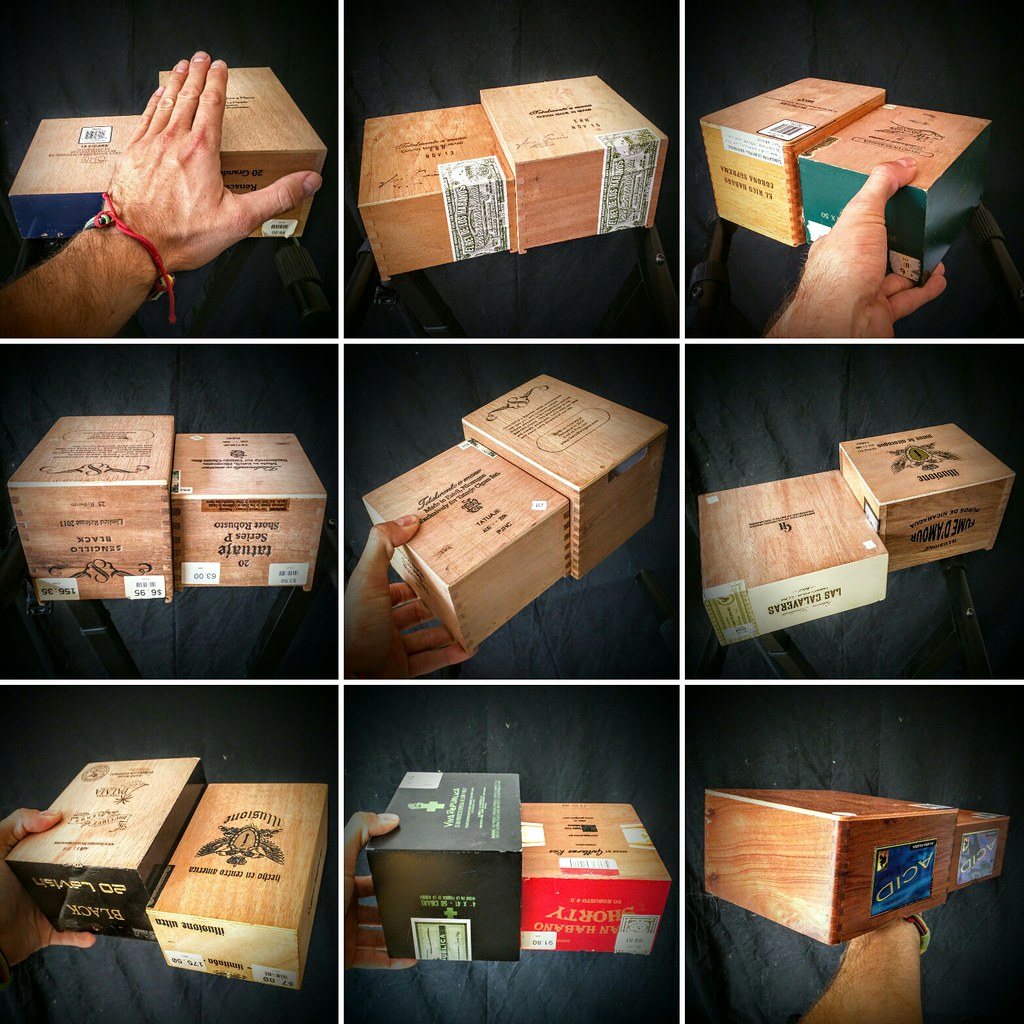The image is composed of a 3x3 grid, totaling nine photographs, each showcasing two cigar boxes against a black fabric background. Most boxes are crafted from bare white pine wood, though some stand out in black, blue, or green hues. Each box features paper labels indicating either the price or the origin of the cigars. Human hands, appearing in six of the nine images, are often shown holding or picking up the boxes, likely to illustrate their size. The boxes, sometimes exhibiting black images or text that are not right side up, vary slightly in size and orientation throughout the photos.